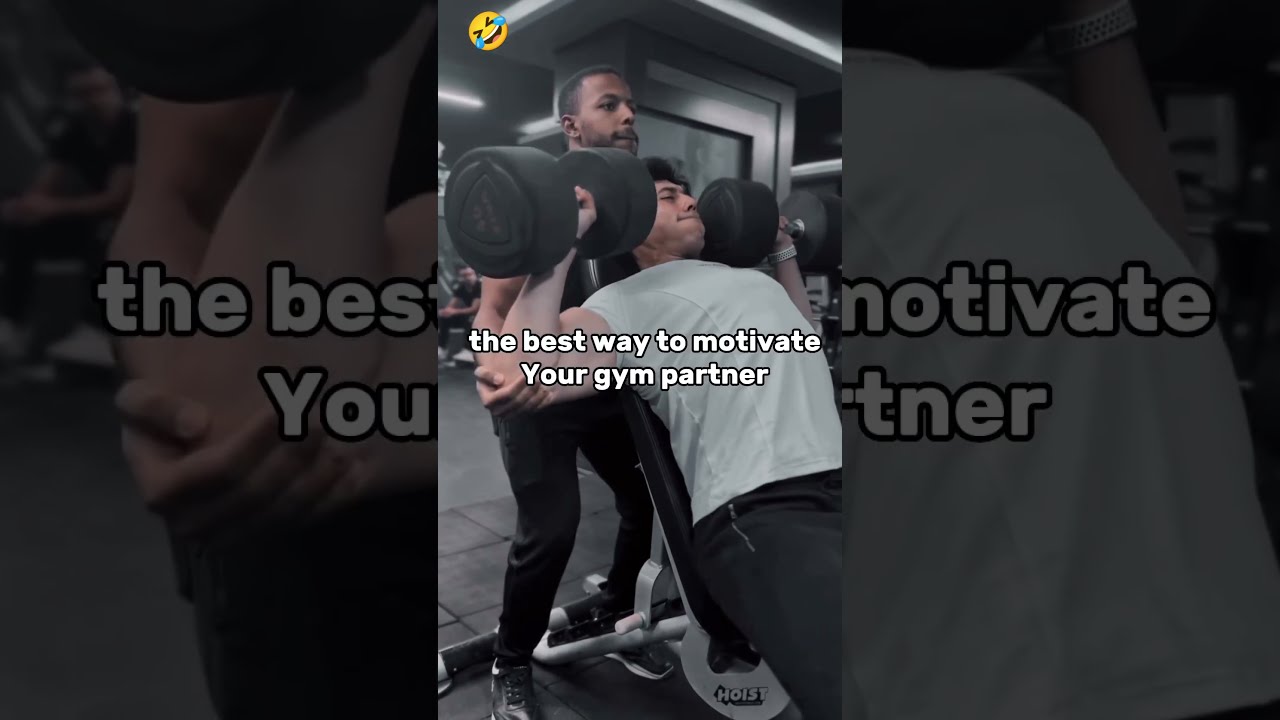This vibrant, portrait-mode image captures a dynamic moment inside a gym. At the center, a man is seated on an upright weightlifting bench, intensely focused on performing shoulder press exercises with hefty black dumbbells. He is clad in a gray short sleeve t-shirt and black bottoms, perhaps sweatpants or shorts. Standing behind him, an African-American man with short hair, a beard, and a mustache is diligently spotting him, hands gently gripping his elbows for support. Both men are bathed in the gym's ambient lighting, highlighting their effort and concentration.

Enhancing the image, bold white text spans two lines across the center, proclaiming, "The best way to motivate your gym partner." A small, jovial emoji depicting a face laughing and crying simultaneously sits in the upper left corner, adding a touch of humor. The entire scene is framed within a larger, darker, landscape image of the same setting, further emphasizing the focused action in the foreground while subtly showcasing the background environment of the gym.